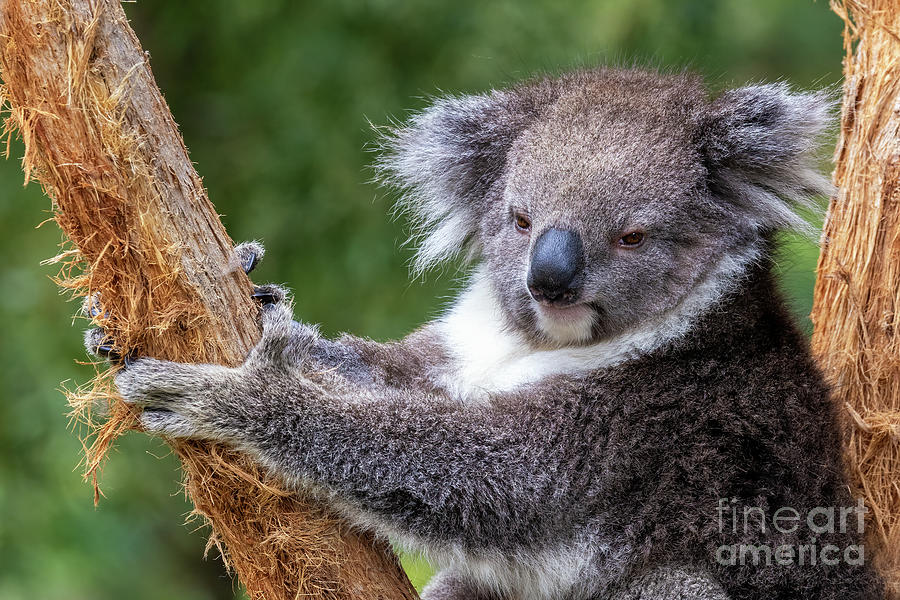In this digital photograph, an elderly koala bear is perched between two partly shredded and whittled-down tree branches, likely worn by the koala’s own claws. The koala, with its arms outstretched, clings to the fuzzy-textured bark of the branch on its left side, bits of wood visibly flaking off. The koala’s fur is an unkempt mix of brownish-gray, with darker shades around its ears and back, and white on its chest, mouth, and the tips of its fuzzy ears. Its large black nose and small brown eyes contribute to its somewhat bored expression. The background features lush, out-of-focus green foliage, enhancing the natural setting. An overlaid text in the lower right corner reads, "Fine Art America."